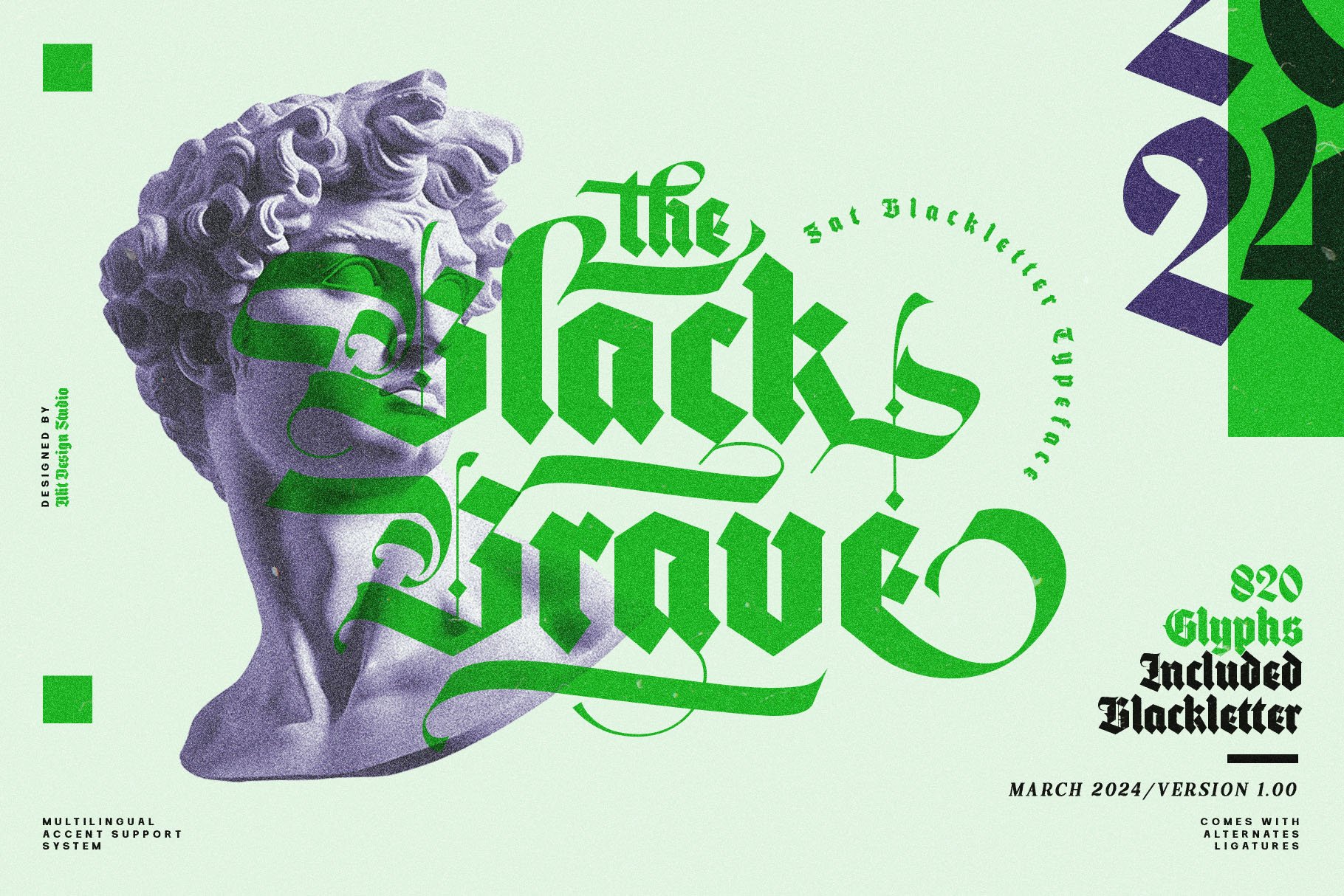The image is a digital art poster featuring a Greek or Italian-style alabaster bust reminiscent of Michelangelo's David, shown from the neck up with curly hair. The bust is rendered in a predominantly black and white with a slight blue filter, positioned on the left side of the composition. Overlaid on the bust is ornate green script that reads "The Black Grave" in the center of the image. The right side of the poster contains additional text in bright green, including "820 glyphs included," "Black Letter," "March 2024 version," and "comes with alternative ligatures multilingual accent support system." There are also some green dots on the left side, enhancing the graphic design. The background is a light shade that appears to be either off-white, blue, or gray, lending a neutral backdrop to the prominent elements of the design. Despite some of the text being illegible, it's clear the poster is a typographic showcase designed by "By List Design Studio."